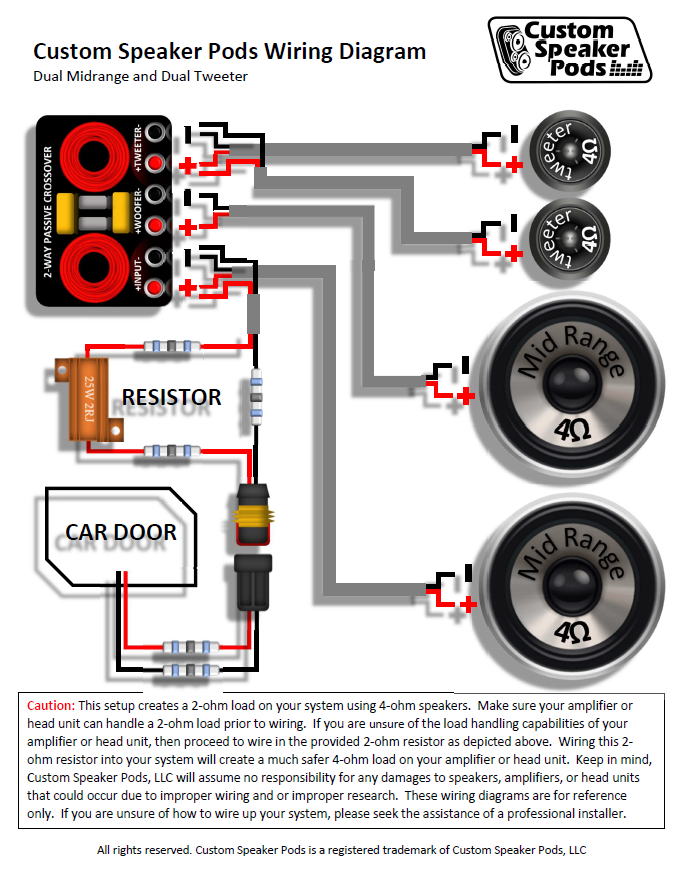The image is a detailed wiring diagram titled "Custom Speaker Pods Wiring Diagram - Dual Midrange and Dual Tweeter," displayed in black text on a white background at the top left. On the top right, another title reads "Custom Speaker Pods," accompanied by a small company logo. The diagram is divided into distinct sections, with the left-hand side illustrating various electrical components, including resistors, controllers, and car door diagrams. These components are interconnected by gray wires, which are marked with red plus signs and black minus signs for ground.

In the right-hand section, the diagram features circular speakers with a metallic-looking center, labeled "mid-range 4 ohms." The wiring is visually tracked from these speakers back to the controllers and resistors. The bottom of the image contains a cautionary note, warning that this setup generates a 2-ohm load using 4-ohm speakers, advising users to ensure their amplifiers or head units can handle the load or to use a 2-ohm resistor to create a safer 4-ohm load. The notice stresses that Custom Speaker Pods assumes no liability for any potential damages due to improper wiring and recommends professional installation for those uncertain about the process.